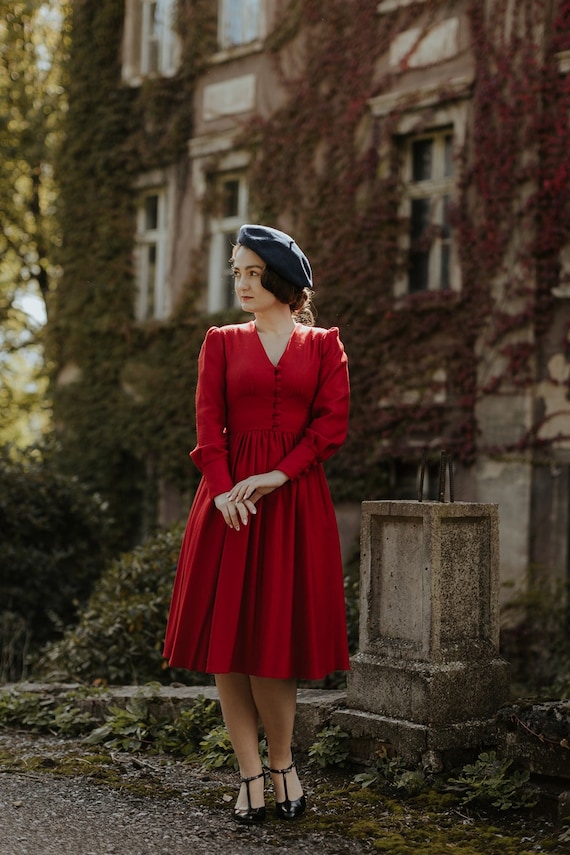This color photograph features a pale-skinned woman in a formal, bright red dress with long sleeves and red buttons down the front, flaring out slightly at the waist. The dress reaches just below her knees and is complemented by her black T-strap heels. Perched at an angle on her head is a dark blue beret. Standing in the street, she looks to her right and touches her right hand with her left, seemingly waiting for someone. Beside her to the right is a stone pedestal with a few bits of rebar sticking out of the top. The background showcases a gray, stone-like house cloaked in lush green vines, with some parts turning red. The house has three visible windows and appears somewhat old-fashioned, partially obscured by the shallow depth of field, which also reveals a sunlit, outdoor scene around the edges of the photograph.